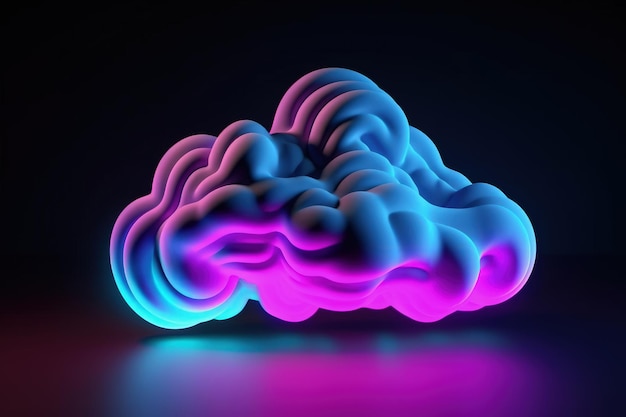A mesmerizing 3D artist rendition depicts a neon-colored, cloud-like structure hovering just above a reflective black tabletop surface. This psychedelic illustration features a blend of soft and vibrant hues: purplish lights and pale grays, alongside neon pinks, blues, and turquoise. The cloud, with an almost toothpaste-like texture and intricate, brain-like lines, is illuminated from below, glowing brightly in magenta and cyan on its underside. Subtle pink highlights accentuate the arches and bubbling top on the left side, while a soft blue light bathes the right side. The entire composition is set against a stark, solid black background, enhancing the luminous and otherworldly appearance of the cloud and its reflection.